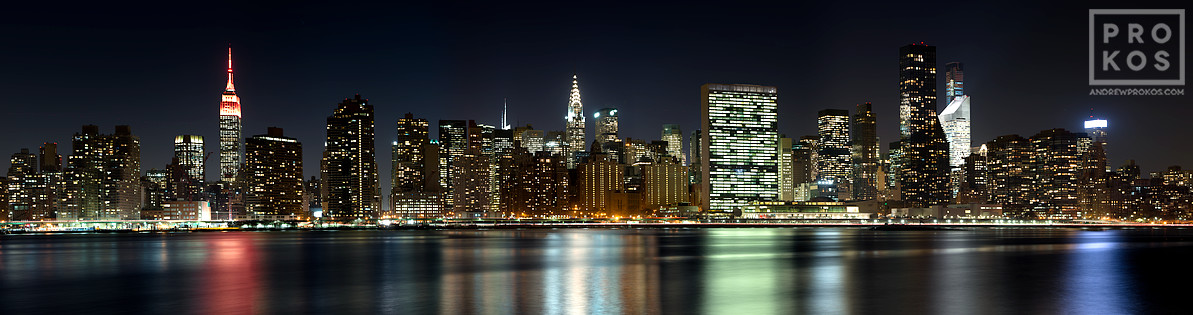The image showcases a panoramic shot of a city skyline, likely at night. Dominating the center is a very tall, wide building adorned with both red and green lights. To its right, there is an unusually shaped building that features a highly illuminated, white triangular top. Further right, one can spot another building with a circular top that glows in fluorescent blue. On the far left, a tall building with a pointed spire is visible, illuminated in orange and white as it ascends.

In the foreground, the city is reflected on a body of water that lies still, capturing the vibrant lights from the skyline in hues of white, yellow, red, and blue. The sky above transitions from dark gray at the top to a slightly lighter shade towards the bottom. The upper right corner of the image bears the watermark "Prokos" and "AndrewProksos.com," indicating the photographer's signature. The overall ambiance of the photo is lively with a striking contrast between the illuminated buildings and the still, reflective water below, creating a mesmerizing nighttime urban landscape.